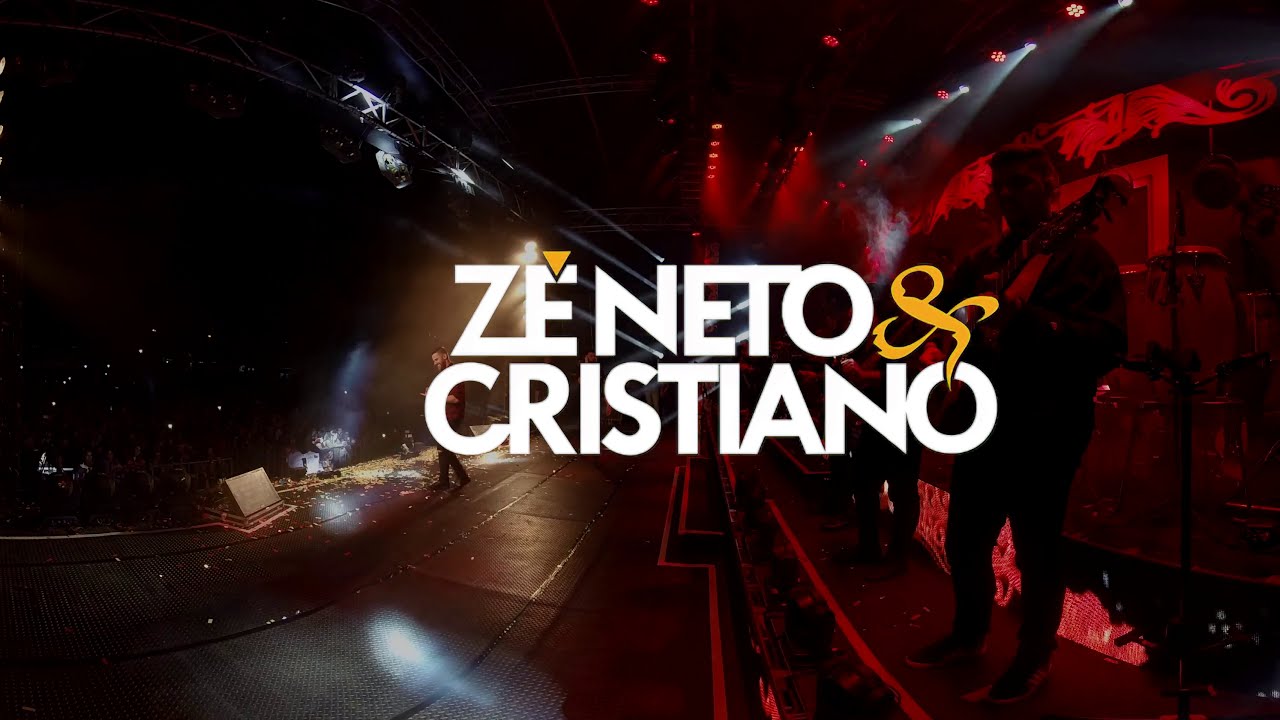This image showcases a musical performance by Zeneto and Cristiano, as indicated by the bold white letters "Z-E-N-E-T-O" and "C-R-I-S-T-I-A-N-O" prominently centered on the screen. The stage is the focal point, taking up about 85% of the image, with minimal visibility of the crowd due to the dark lighting. Two musicians dominate the stage: one in the foreground, under bright stage lighting, possibly singing amidst some confetti, and another towards the back, playing a guitar, backlit with red lights. The stage itself is mostly black, with overhead lights creating a dynamic atmosphere of red and black hues. Though faint, the distant crowd can be partially discerned, suggesting the performance is taking place in a large auditorium packed with spectators.